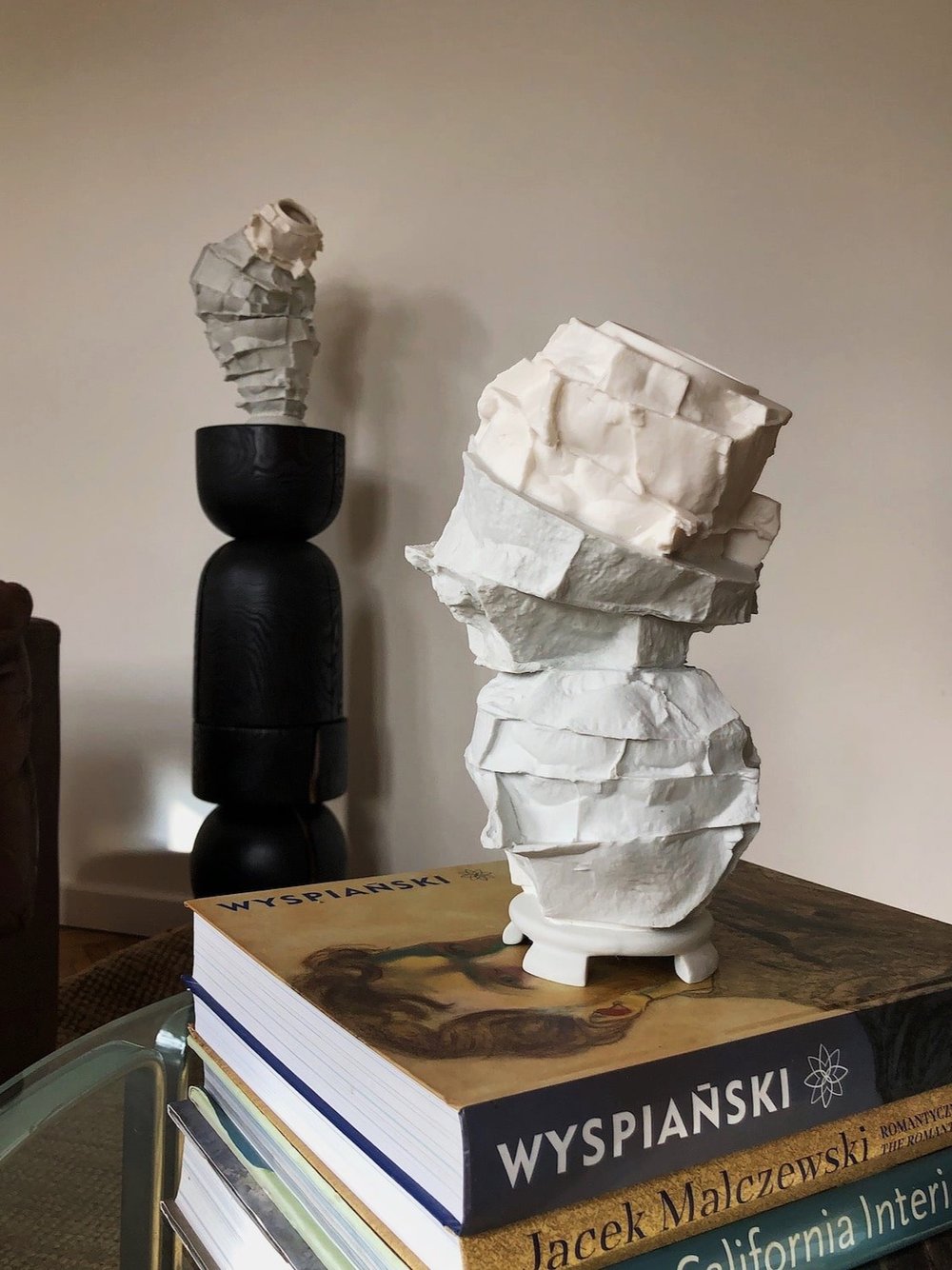The photograph captures an interior setting, likely in someone's home, showcasing two distinct and intriguing clay statues. The backdrop is a well-lit room with a warmly painted light brown (or beige) wall, complemented by white trim along the baseboards. In the lower right corner of the image, there's a dark table upon which several literature-focused books are stacked. The books, primarily brown and black, include titles such as "Wyspianski," "Jaquique Malkuszynski," and a partially visible one that appears to be "California Interiors."

The clay statue on the left is positioned on an interesting, artistic black pedestal which resembles a lipstick-shaped cylinder split and rearranged into a unique form. This statue, beige and tan in color, consists of assorted angled clay sections that don't quite align, creating a somewhat unbalanced and abstract appearance. The intricately designed pedestal adds to its artistic allure, with elements described as a bowl part and a middle cylinder, enhancing its sculptural depth.

On the right side, another compelling statue is predominantly white with a tan top, situated on the aforementioned stack of literature books. This sculptural piece appears layered with what might be white papier-mâché or carved plastic, creating a striking contrast against the dark table and books. Its form is somewhat snowman-like, featuring a man's face with a long, pointed nose, apparently blindfolded, and capped with a flat top. Above the stacked books, this statue seems to loom with a whimsical yet solemn presence.

Together, these elements present a vivid tableau of abstract art within a thoughtfully appointed living space, bordered by the edge of a couch and possibly a glass coffee table spotted at the corner of the photograph.